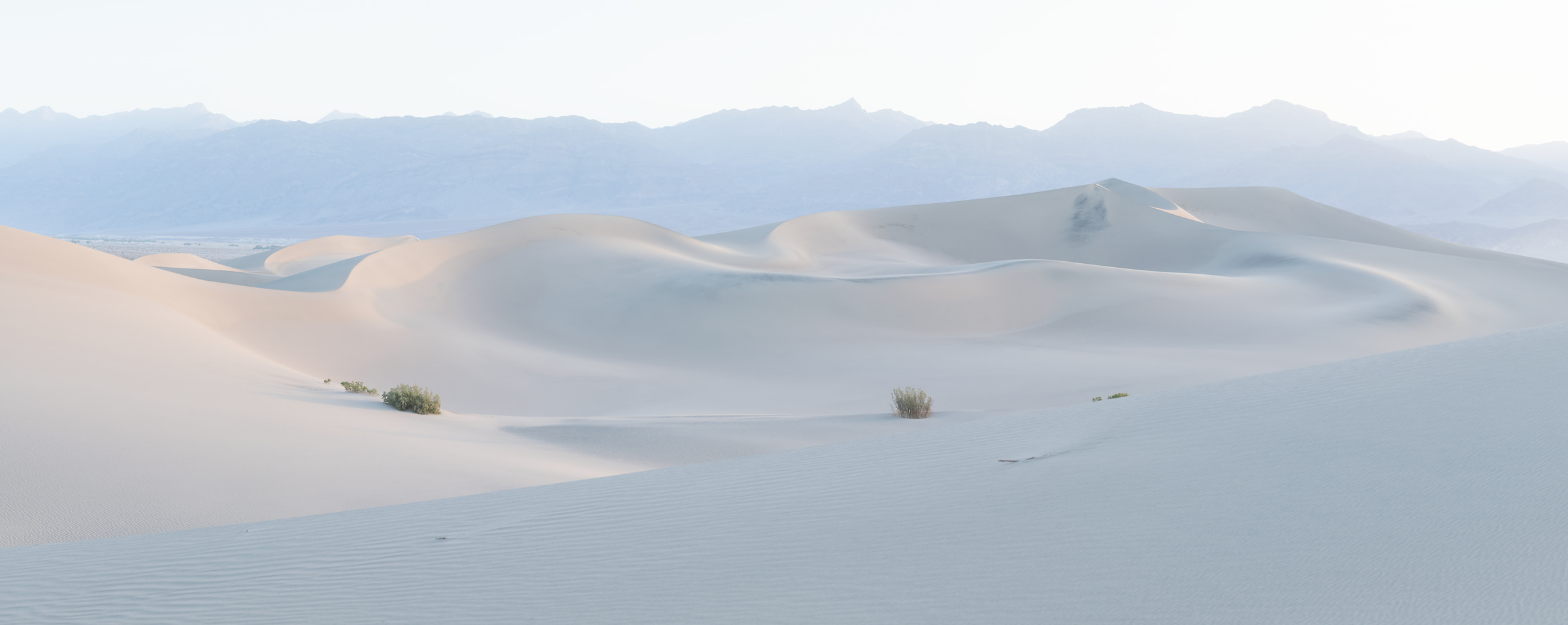The image presents a vast, ethereal landscape dominated by a white theme, making it challenging to discern whether it's a photograph or a painting. The foreground features sweeping white mounds that resemble either snowy drifts or sand dunes, possibly hinting at a location like White Sands. These mounds are accented by a few tufts of desert scrub grass or small green plants poking through. Shadows are cast from the right, indicating the sun's position, and giving the dunes a darker tone on their left sides.

In the distance, the landscape blurs into a faint silhouette of a mountain range that appears almost gray, blending seamlessly into an almost white sky with just a hint of light blue. The background is foggy or perhaps washed out, further enhancing the surreal, monochromatic quality of the scene. The overall impression is one of purity and starkness, with the mounds of white sand or snow creating gentle, undulating swirls across the terrain.